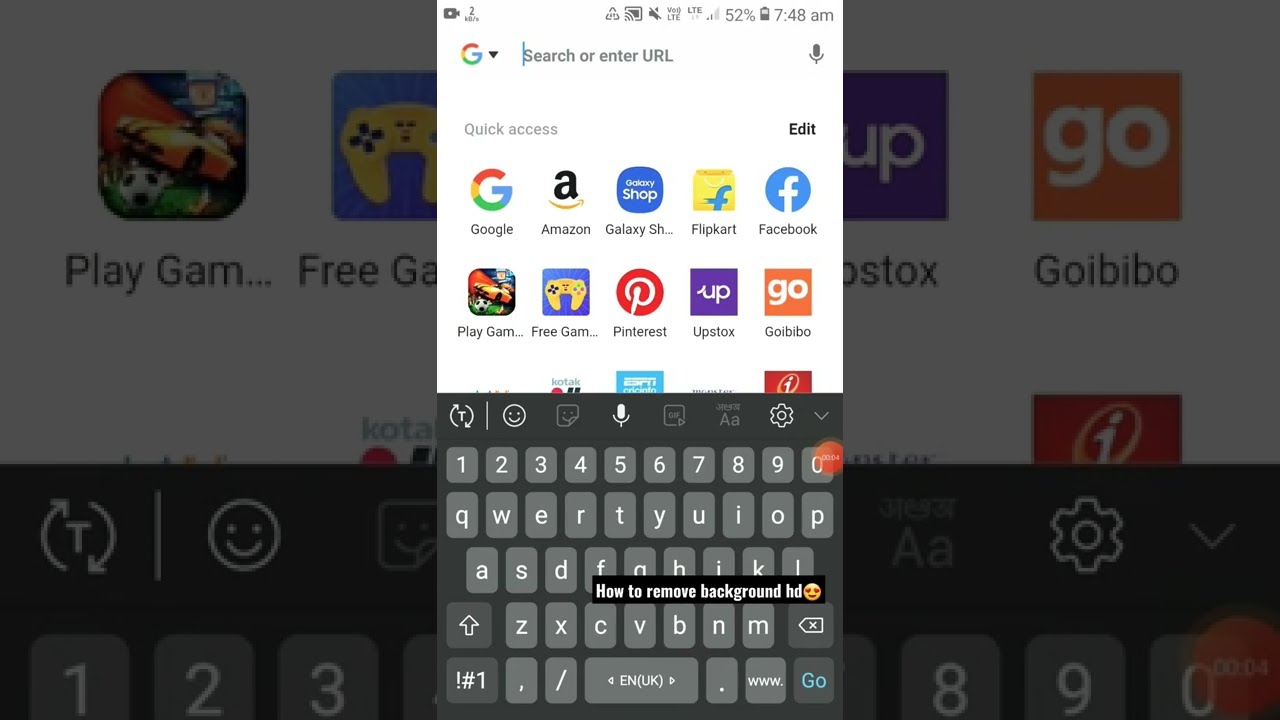This is a detailed screenshot of a smartphone, specifically an Android or Galaxy device, displaying the Google search bar at the top with the Google icon and the ‘Search or Enter URL’ field, followed by a microphone icon on the far right. The screen is in light mode with a white background. Below the search bar, there’s a section labeled 'Quick Access' featuring various app icons with their respective logos: Google (a multicolored ‘G’), Amazon (an ‘A’ with an arrow), Galaxy Shop, Flipkart, Facebook (a white ‘F’ on a blue background), Play Games, Free Games, Pinterest, Upstox, and Goibibo. The bottom portion of the screenshot prominently displays the device’s gray QWERTY keyboard. Superimposed over the keyboard, in a black background with white text, is a caption reading "How to Remove Background HD," accompanied by a smiley face emoji with hearts for eyes. The left and right panels of the image seem to be magnified sections of the main screenshot, highlighting specific details like the top numbers on the keyboard and parts of the Goibibo app icon.